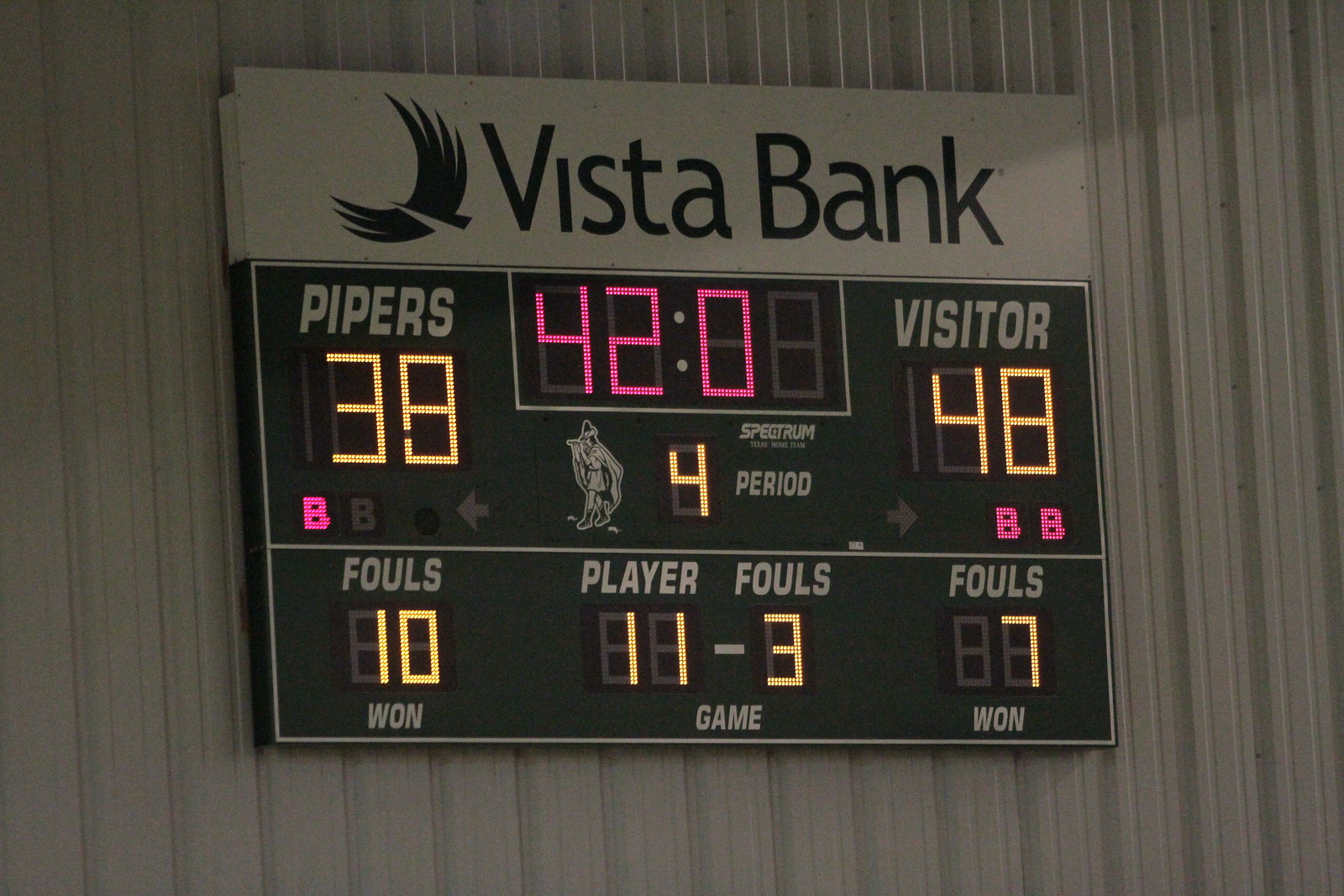The photograph captures an intricate electronic scoreboard mounted on a white, corrugated metal wall. At the top of the scoreboard, the name "Vista Bank" is displayed prominently in black text next to a stylized logo of a flying bird. The scoreboard is divided into three main sections. On the left, the word "Pipers" is written in white text over a green background with a score of 38 in orange LED lights beneath it. Below the score, a pink LED light forms the letter 'B' and nearby, the word "Fouls" with the number 10 in gold LED lights. 

The central section features a clock or timer display in pink LED lights showing "42-0," indicating a possible period marked as '4.' To the left of this pink display are additional white LED indicators showing the game's progress and metrics.

On the right section, the word "Visitor" is displayed in white text with a score of 48 in orange LED lights below it. Beneath the score, two 'B's' are lit in pink LED lights. In this section, the word "Fouls" appears again with a gold LED number 7 beneath it. 

Combining the repeated elements and shared details from all captions, this scoreboard effectively balances team scores with additional metrics, expertly integrating visual elements and text to communicate game information.